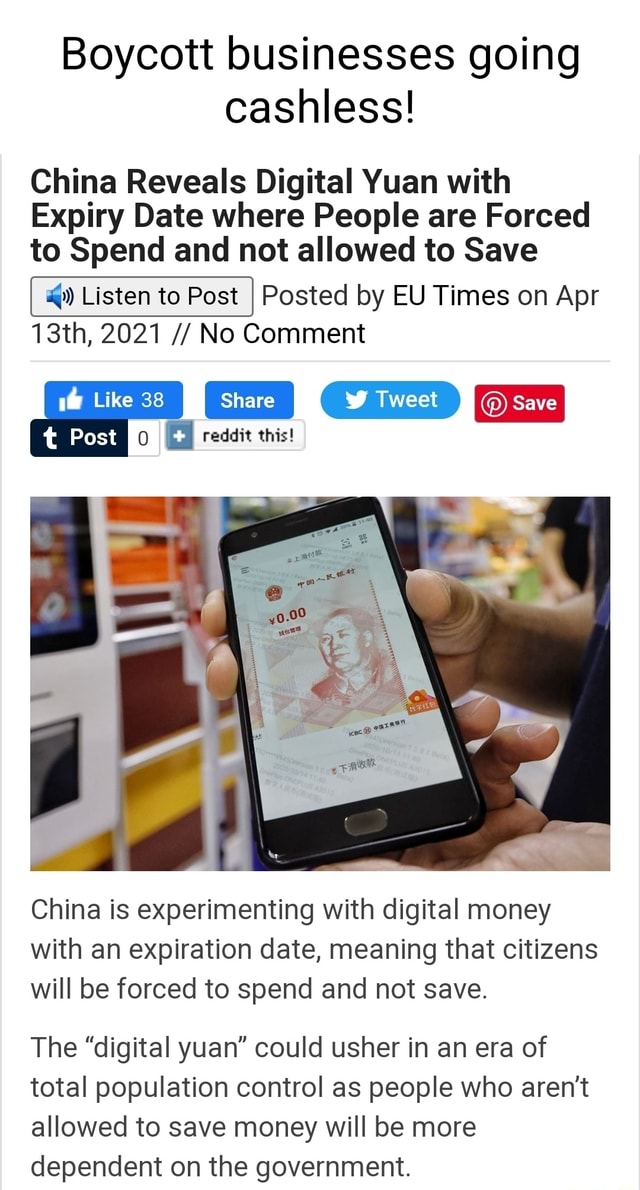**Caption:**

At the top of the image, bold black text reads, "Boycott businesses going cashless." Below this, in prominent bold text, a headline states, "China reveals digital yuan with expiry date where people are forced to spend and not allowed to save." Adjacent to the text is a small microphone icon with the label "Listen to post," indicating an audio version of the post is available. 

Further down, the post is credited to EU Times, dated April 13th, 2021, and marked with "no comment."

The image features several interactive buttons:
- A like button with a white thumbs-up icon and the number 38.
- A blue "Share" button.
- A Twitter share button with the label "Tweet" and a bird icon.
- A red Pinterest save button labeled "Save."
- A button labeled "T post 0."
- A button labeled "Reddit this."

Below these buttons is an image showing someone holding up a phone displaying what appears to be digital currency information.

Underneath the image, a paragraph explains that China is trialing digital money with an expiration date. This new form of currency will force citizens to spend instead of saving, potentially increasing dependency on the government and leading to greater population control.